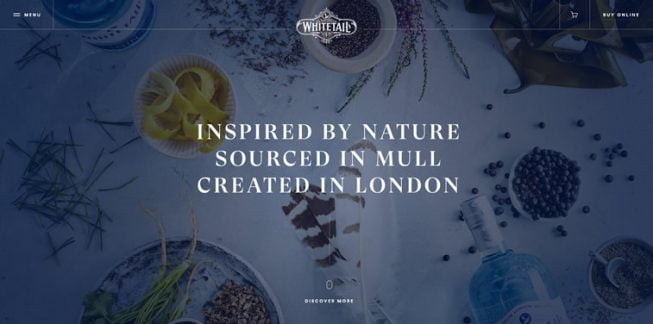This image is a horizontal screenshot with a translucent dark bluish-purple overlay. At the center of the image, bold white text in three lines reads: "Inspired by Nature, Sourced in Mole, Created in London." The top center of the image features the company's logo, "White Tail," indicating that this is a gin company.

In the lower center, very small white text reads "Discover More," inviting viewers to explore further. The image additionally has a small menu toolbar located in the upper left-hand corner, and in the upper right-hand corner, there are icons for shopping and an option to "Buy Online."

The background photograph beneath the translucent overlay shows an elegantly arranged assortment of ingredients and objects. Central to the image are feathers adding an artistic touch. In the lower left quadrant, there is a bowl containing food, possibly featuring a circular rind that resembles lemon. An additional bowl with berries and the top of a gin bottle, along with a scoop filled with some type of grain, are positioned in the lower right-hand quadrant. Additionally, a bottle can be seen in the upper left-hand corner of the image. This composition reinforces the natural and high-quality ethos of the White Tail gin brand.